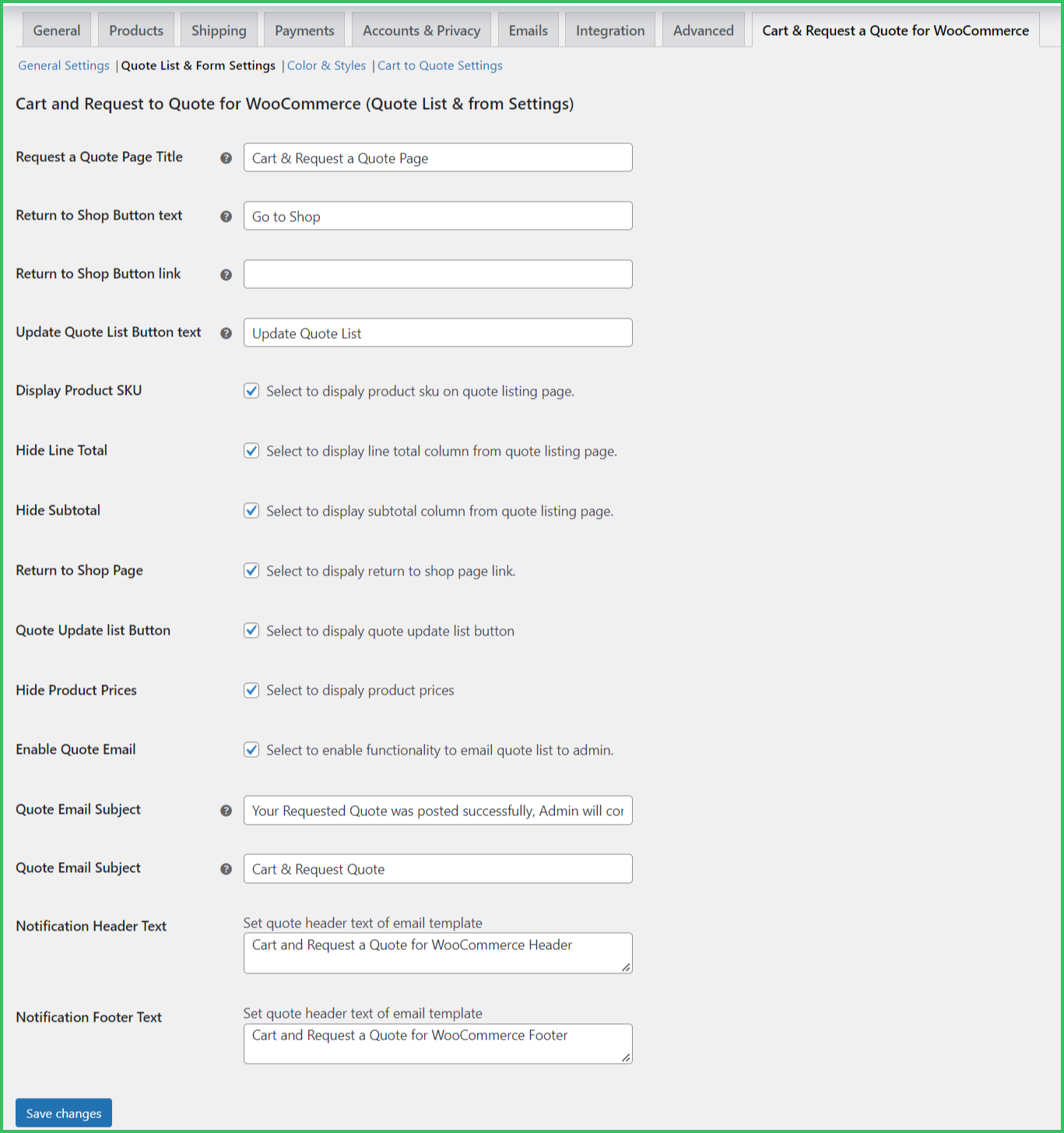The image features a gray background outlined in green, displaying various general product settings for a WooCommerce platform. Specifically, it includes sections for shipping, payments, accounts and privacy, emails, and integration advance. 

In blue text, it identifies "general settings" for cart and request features, as well as a quote request system for WooCommerce. Below it, there are settings for quote lists and form settings, colored in blue. Additionally, there's a segment labeled "Cart to Quote Settings" that pertains to quotes and cart functionalities for WooCommerce.

Prominently, it has a section titled "Request to Quote" with a page title. A black circle with a white question mark is visible, which likely indicates help or additional information. There are also buttons for "Request to Shop" with corresponding question marks for guidance and a "Return to Shop" button link, also with a question mark enclosed in a box.

The scene showcases text for updating quote lists, with selected boxes to display product SKUs and a selection to enable the display of product SKUs on the quote listing page. Every box in the image appears to be selected, ensuring full visibility of product details in the quote listing feature.